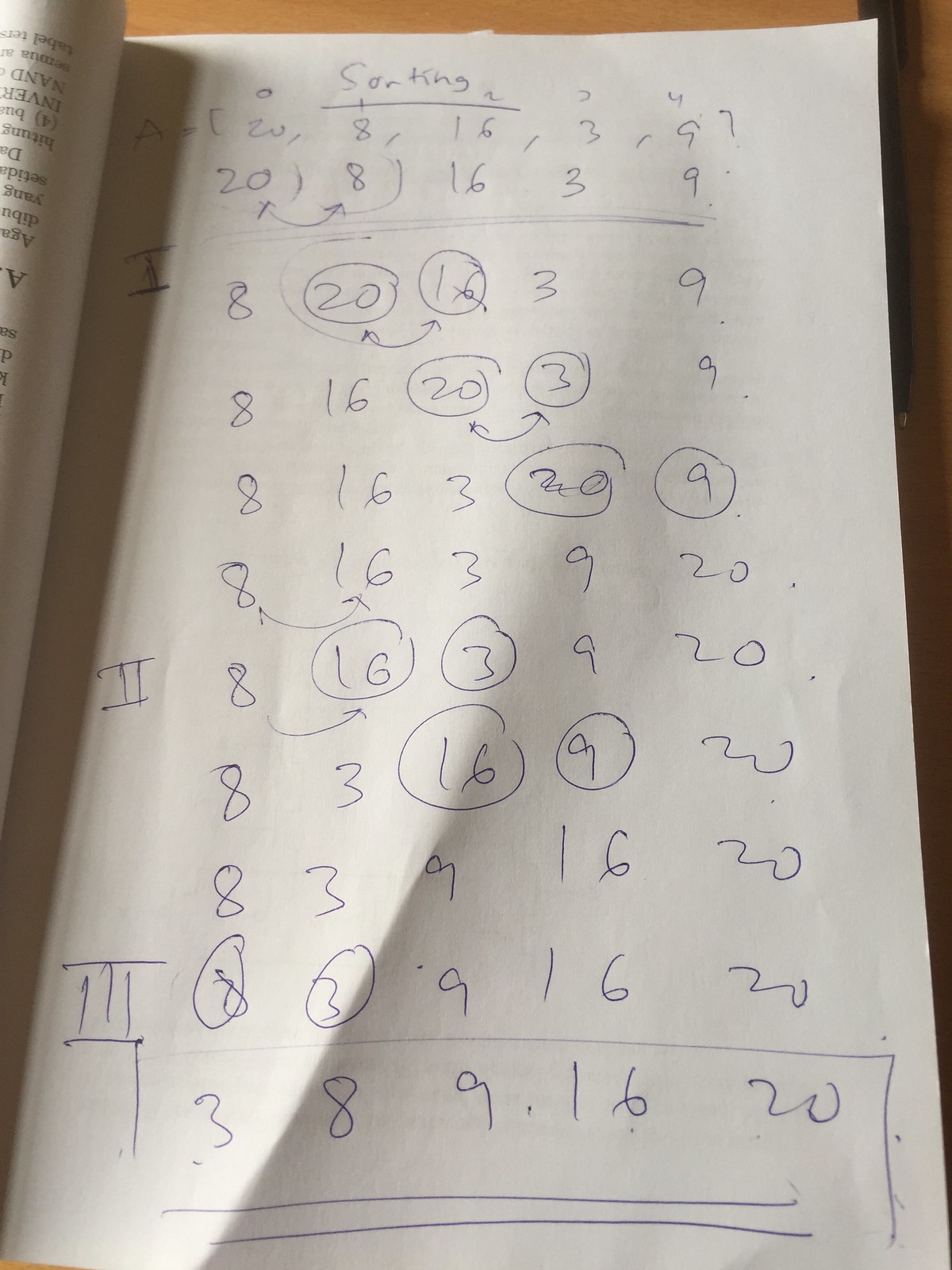Close-up of a Book Page, Annotated with Handwritten Notes: A high-resolution image captures a close-up view of an open book or magazine, focusing specifically on the right-hand page. The visible page features handwritten notes, jotted down in either a dark blue or black pen, detailing a sorting algorithm. The printed text on the page is titled "Sorting," followed by an array of numbers arranged in a matrix-like format. The initial sequence of numbers is: 20, 8, 16, 3, and 9. The handwritten notes systematically outline a nine-step algorithm, illustrating the process of sorting these numbers in ascending order. The steps are clearly labeled from 1 to 9. By the final step, the numbers have been successfully sorted into the sequence: 3, 8, 9, 16, and 20. The detailed annotations provide a step-by-step guide to understanding the sorting algorithm and its functionality.